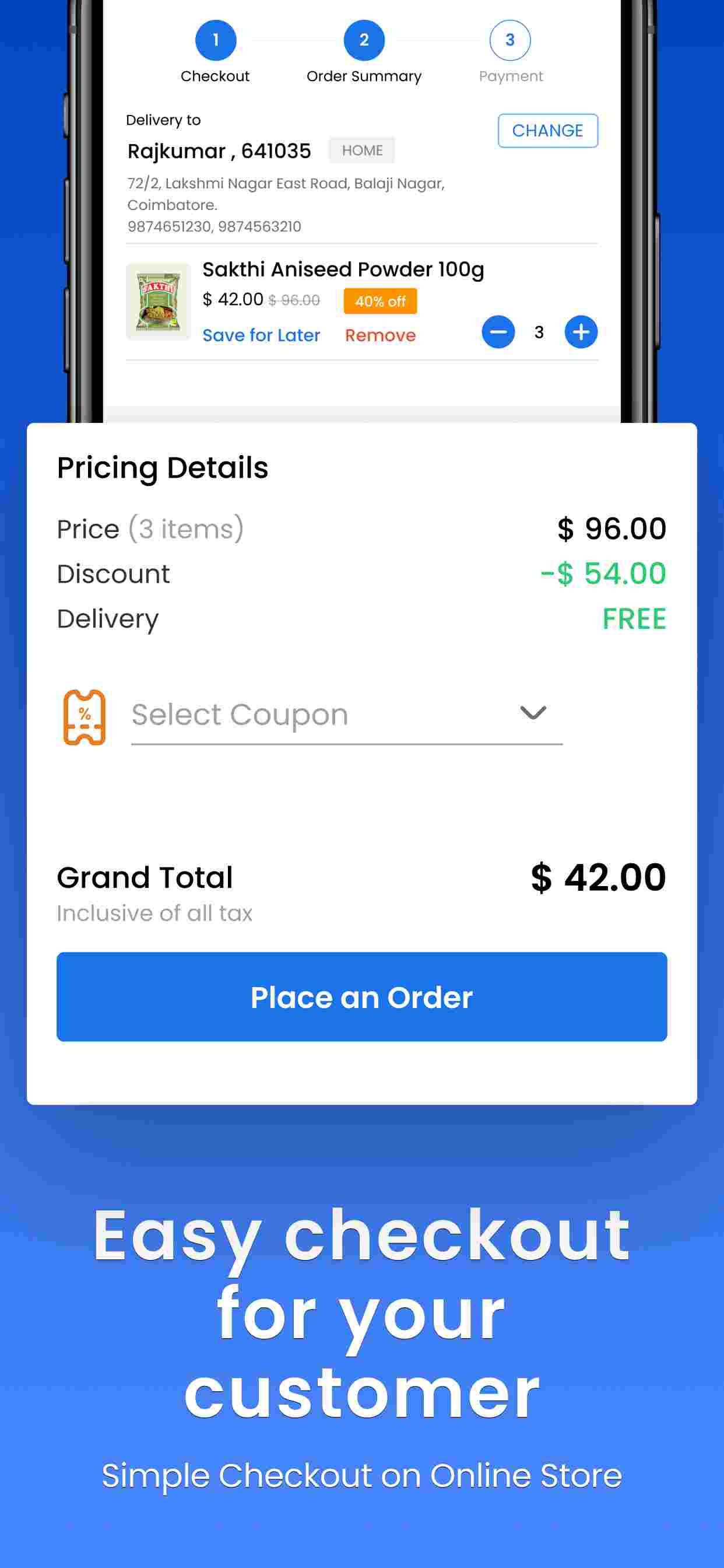This image serves as a promotional visual for an online store, emphasizing the simplicity of their checkout process through their mobile app. The focal point is a smartphone, displayed centrally but partially cropped, with the top and bottom sections not visible. Overlapping the lower part of the phone screen is a white pop-up box. 

On the top left corner of this box, the heading reads "Pricing Details." Below this title is a breakdown of costs: "Price," indicating the total for three items, listed as $96. Subsequently, a line indicates a "Discount" of $54, visually marked as a deduction. Further down, "Delivery" is noted, stated to be free of charge. 

A dropdown menu option invites the user to "Select Coupon," providing a potential for additional savings. At the bottom of the white box, it prominently displays the "Grand Total," inclusive of all taxes, calculated to be $42. This detailed composition underscores the streamlined and user-friendly checkout experience provided by the app.